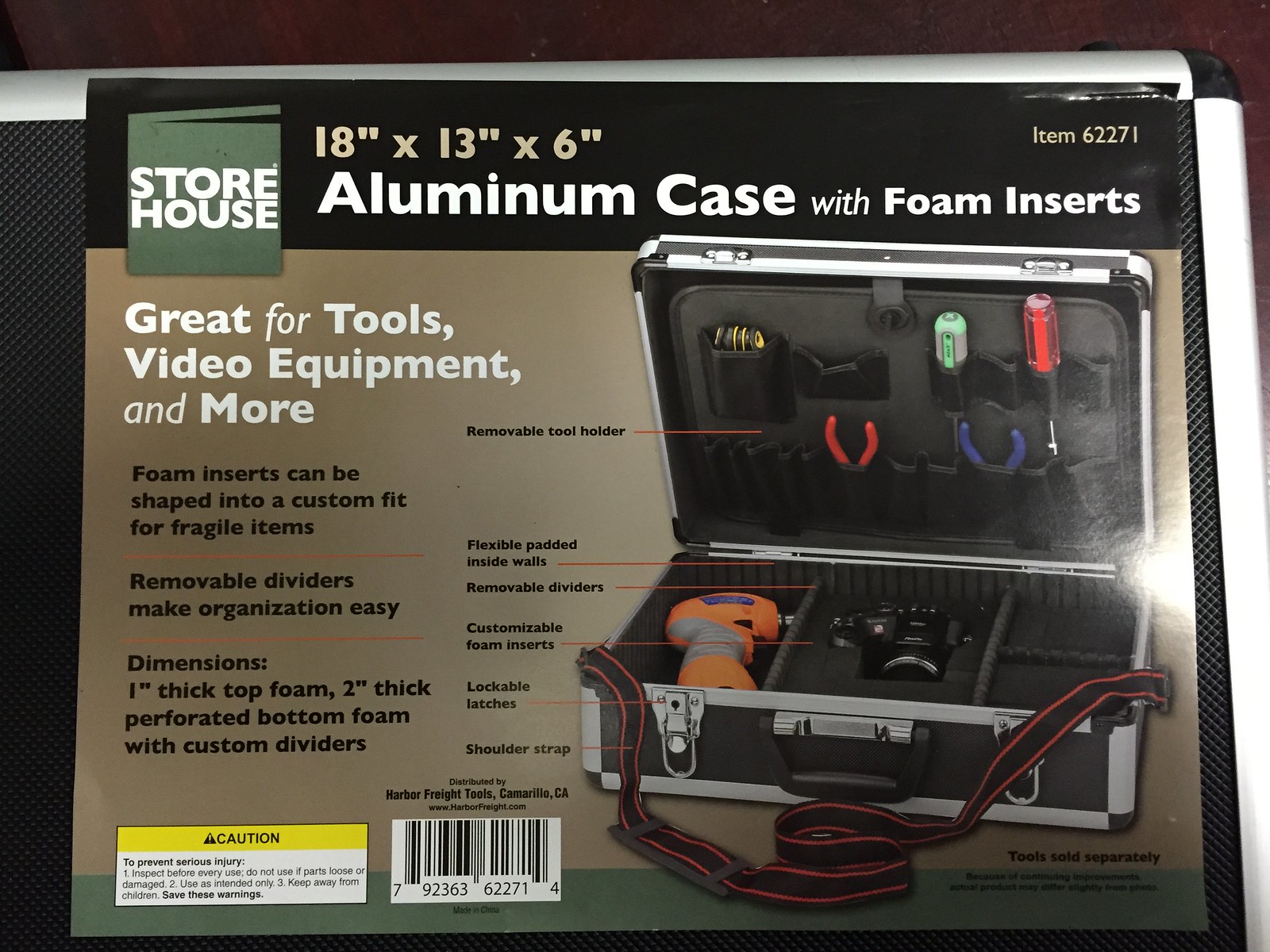This image showcases an aluminum case product by Storehouse, featuring a detailed descriptive paper covering. Prominently positioned on the front, the text "Storehouse" appears in white within a green box in the upper left-hand corner. Adjacent to this, also in white, the dimensions are listed as "18 inches x 13 inches x 6 inches" above the phrase "aluminum case with foam inserts." In the upper right corner, "item 62271" is displayed against a black background.

Center stage on the covering is a picture of the aluminum case itself, boasting a black interior and a silver border. The image depicts various tools neatly organized within the case, which includes a shoulder strap for added convenience. Accompanying the picture, red lines annotate features of the case, highlighting how the foam inserts can be custom-shaped for fragile items and the removable dividers for easy organization. The text elaborates on the interior, noting a one-inch thick top foam and a two-inch thick perforated bottom foam with custom dividers.

At the bottom left, a caution symbol and a black and white barcode (UPC symbol) are present. The overall design and text emphasize that this case is ideal for storing tools, video equipment, and more.